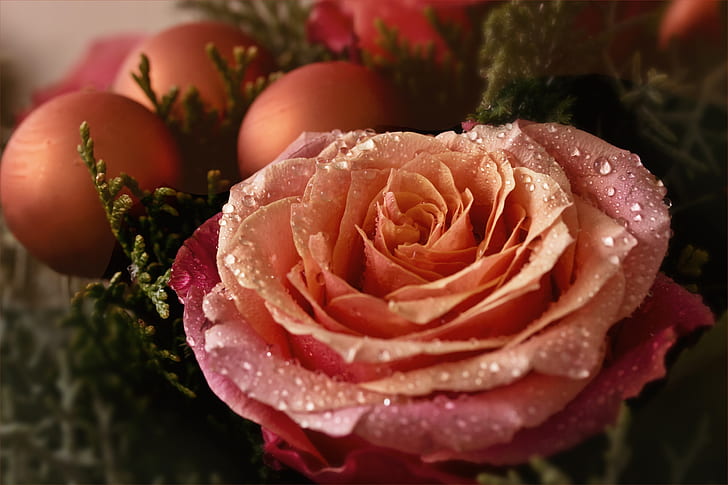The image is a detailed, close-up color photograph of a light pink rose adorned with clear water droplets, resembling tiny ornaments. The rose, off-center and positioned slightly to the right, is surrounded by green branches or needles, possibly from a hedge or evergreen plant. The soft green needles frame the rose, adding to its delicate appearance. The scene has three red balls in the upper left-hand corner, similar in color to the rose, enhancing the festive, wreath-like arrangement. The photo is taken from a diagonal angle with light coming from the upper left, casting gentle highlights and shadows, giving the image a subtle, ethereal quality. The background features a blurry mix of greenery and grayish hues, adding depth to the composition while keeping the focus on the pink rose and its dewy adornments.